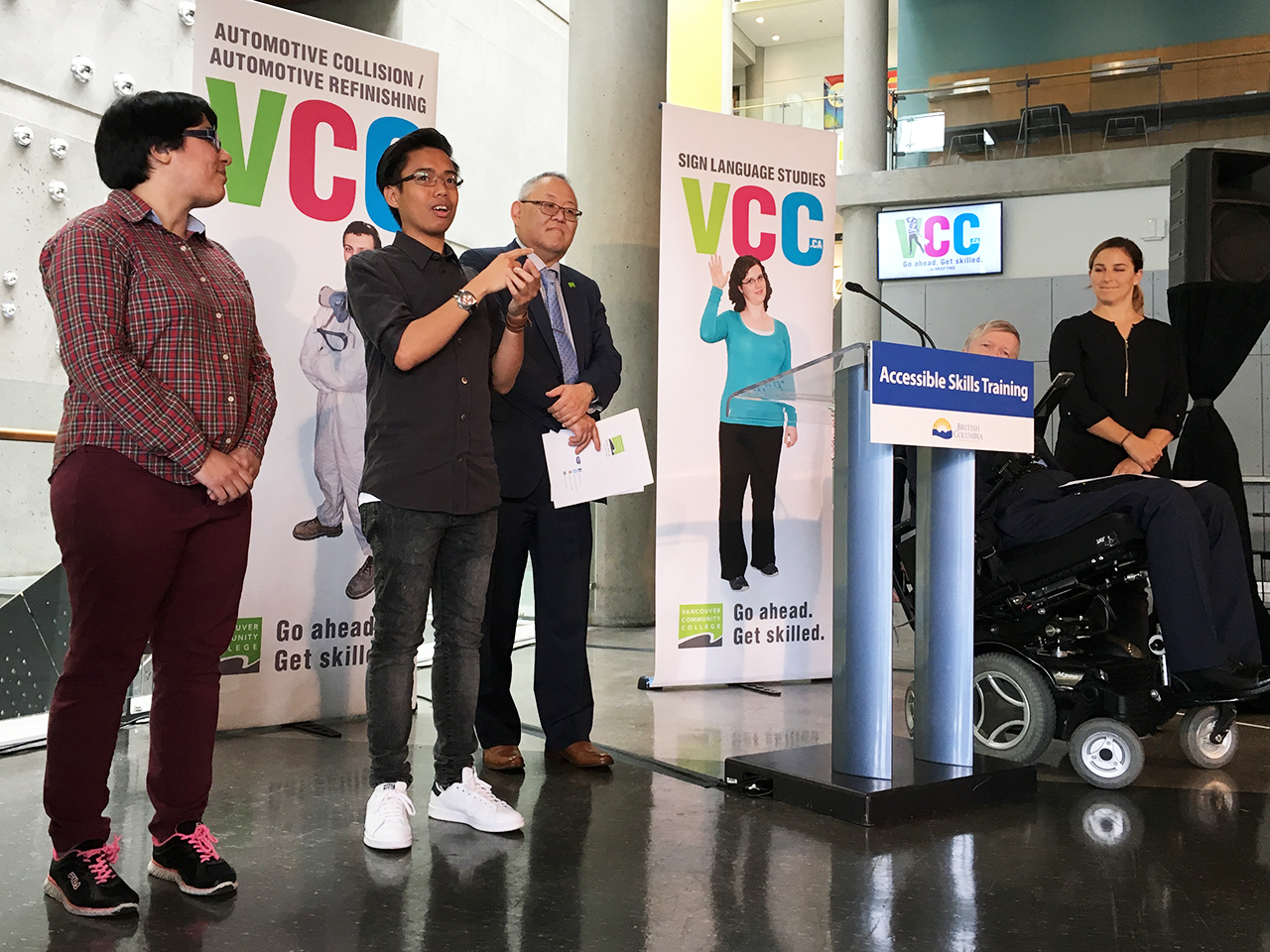In this detailed photograph, a group of individuals is gathered in a convention hall or possibly the large lobby of an office building, engaged in a presentation related to accessible skills training. Central to the scene is a sleek podium with a black base, silver posts, a clear glass top, and a sign that reads "Accessible Skills Training" in blue with white text. Although no one is standing directly behind the podium, a young male speaker, wearing a black short-sleeved shirt, black denim jeans, white sneakers, and glasses, is positioned to the right of the podium. He is actively gesturing with his hands, addressing the audience.

To the young man's right, a female dressed in a maroon shirt and pants listens attentively. On his left stands an older gentleman, likely in his 60s, clad in a blue suit and tie, holding some papers. Further left of the podium, there appears to be a partially visible individual in a tilted-back wheelchair, dressed in a blue suit. Standing next to this individual is a woman in a black outfit, who is smiling and looking towards the speaker.

Behind the group are several posters promoting various skill training programs, including "Automotive Collision / Automotive Refinishing" and "Sign Language Study," both with the tagline "VCC - Go Ahead, Get Skilled." The floor underfoot is a hard, glossy surface, possibly polished concrete. This diverse group, comprising people both standing and in wheelchairs, is clearly involved in an event focused on accessibility and skill development, potentially hosted by a college or technical institute.